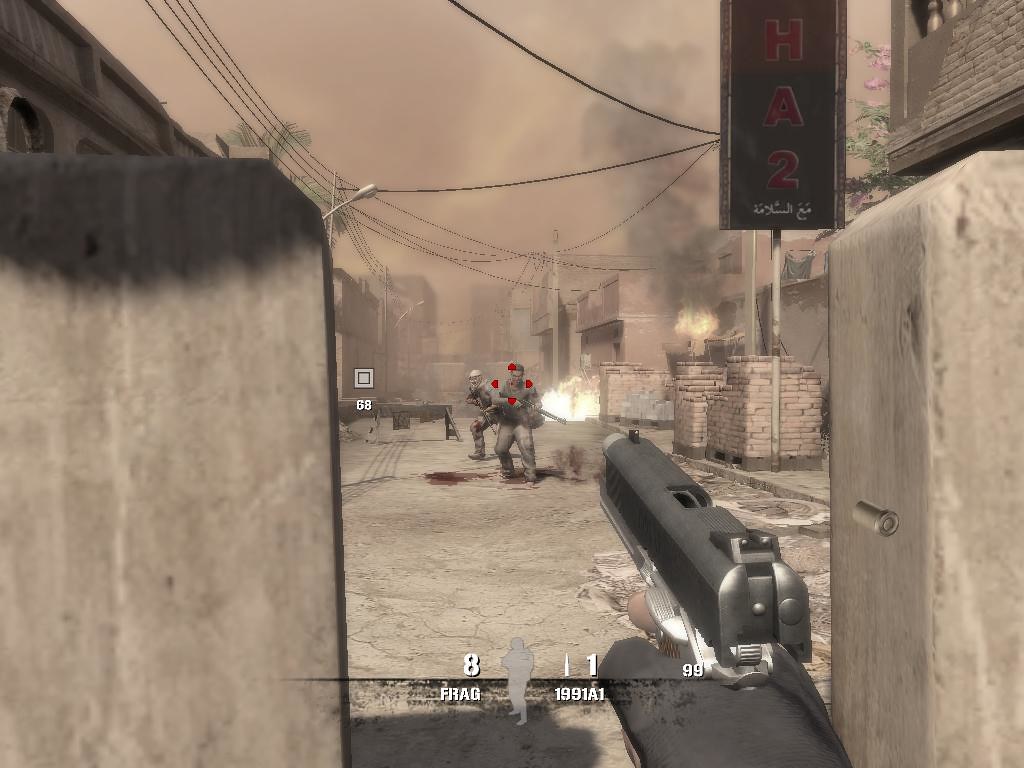This image is a computer-generated screenshot from a first-person shooter video game, depicting an intense urban warfare scene. The vantage point is the player's perspective, showcasing a gloved hand holding a handgun poised to fire. The environment is an Arab city engulfed in chaos, characterized by low brown buildings, brick walls, and a maze of electric wires suspended between structures. A pervasive pinkish-gray smoke cloaks the sky, contributing to the eerie ambiance. The streets, littered with debris and smeared with blood, hint at prior violence. Off in the distance, two soldiers with military rifles, wearing camouflage gear, stand ready with weapons raised, framed by burning buildings. Red target indicators hover around them. Visual details like a gray box with the number 68, game stats such as "8 FRAG, 1991 A1," and the outline of a man indicating health status are displayed at the bottom of the screen. The overall scene suggests a war-torn environment rife with danger and destruction.